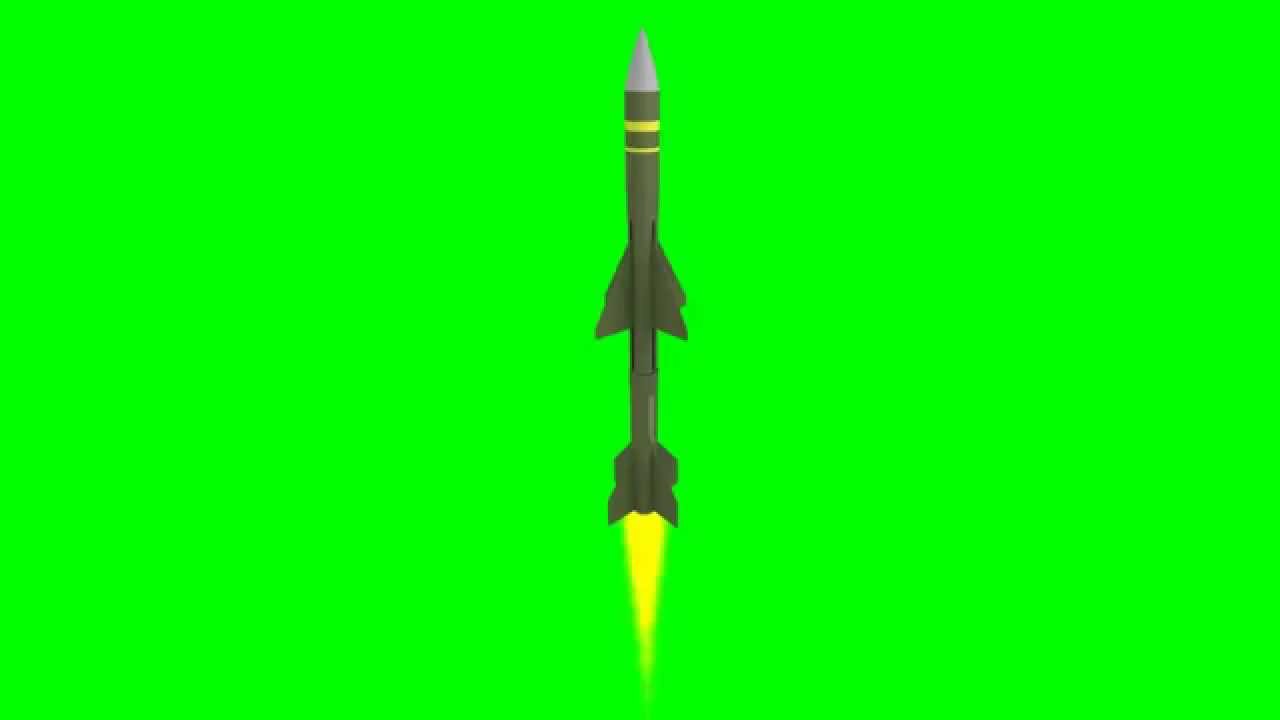The image features a striking, solid bright neon lime green background, free of any design or pattern. In the center of this vivid backdrop, a rocket ship is depicted in flight, with a detailed drawing showcasing its various features. The rocket's body, predominantly a dark gray or military green, sharply contrasts with the neon green background, highlighting its form. The top of the rocket is distinguished by a light gray cone or tip pointing upwards. Just beneath this tip are two prominent stripes: a thin white stripe and a thicker yellow stripe.

The rocket is equipped with multiple fins. There are two larger, triangular fins situated midway on either side of the body, aiding its flight. Additionally, at the bottom of the rocket, there are four smaller, squared fins, with two protruding towards the viewer and two pointing towards the back. The rocket's propulsion is depicted as a pointed yellow flame emanating from its base, signifying its takeoff. Overall, the vivid contrast between the rocket's dark hues and the neon lime green background make the image striking and easily discernible.